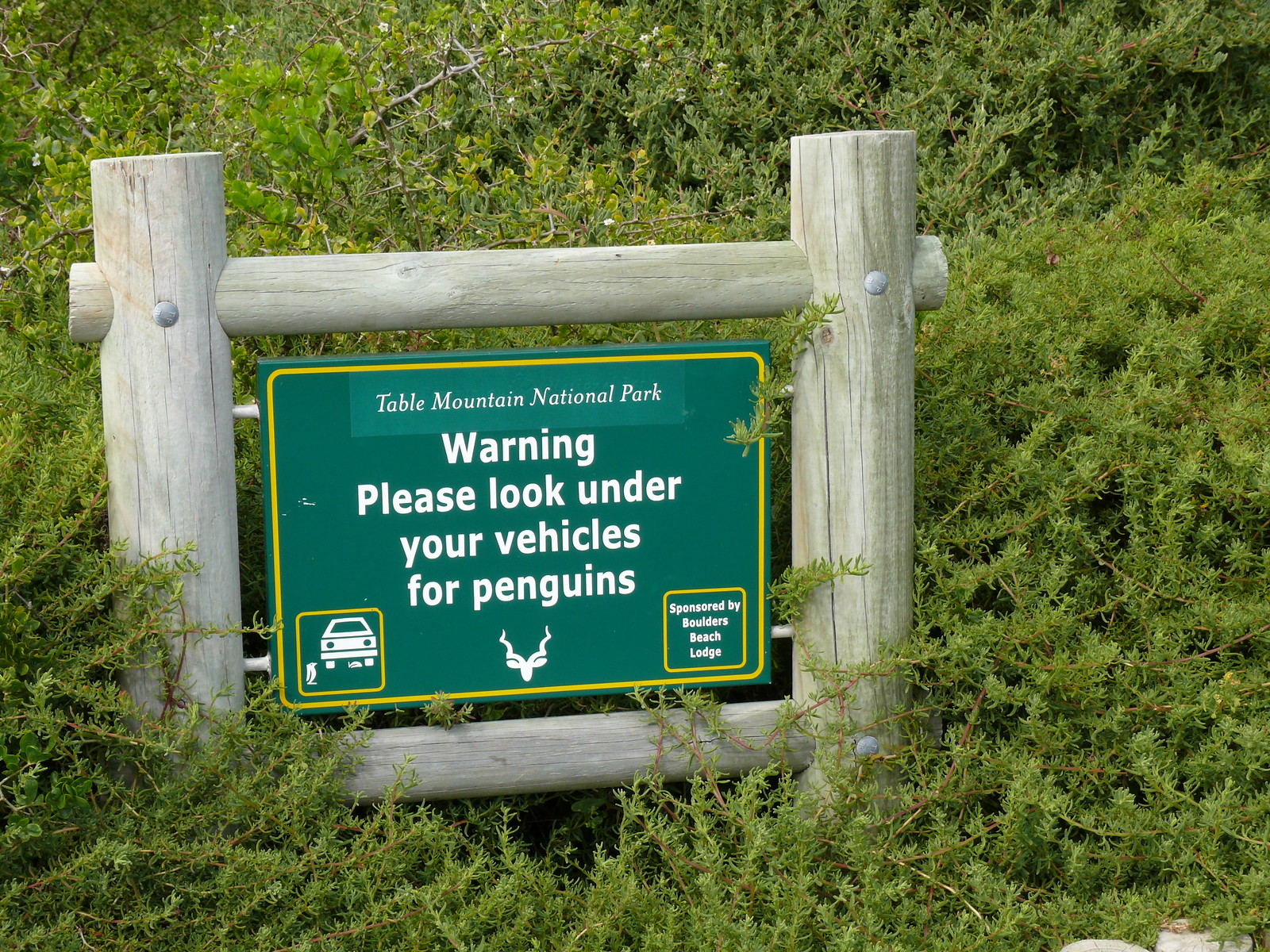In this photograph, we see a lush green field scattered with vibrant plants, and prominently positioned in the middle is a well-constructed wooden frame supporting a warning sign. The frame is fashioned from four large circular wooden posts, forming a square-like structure. The sign inside this frame has a green background and is bordered in a bright yellow color. The central part of the sign features white text that reads, "Table Mountain National Park. Warning, please look under your vehicles for penguins."

Below this main text, there is a white silhouette of an animal resembling an antelope. To the bottom left of the sign, there is a depiction of the back of a car with a penguin underneath it and another penguin standing beside it. On the bottom right, within a yellow outlined square, is the text "Sponsored by Boulders Beach Lodge." The wooden base of the frame is light brown and blends naturally with the surrounding green foliage, adding to the aesthetic appeal of the scenery.